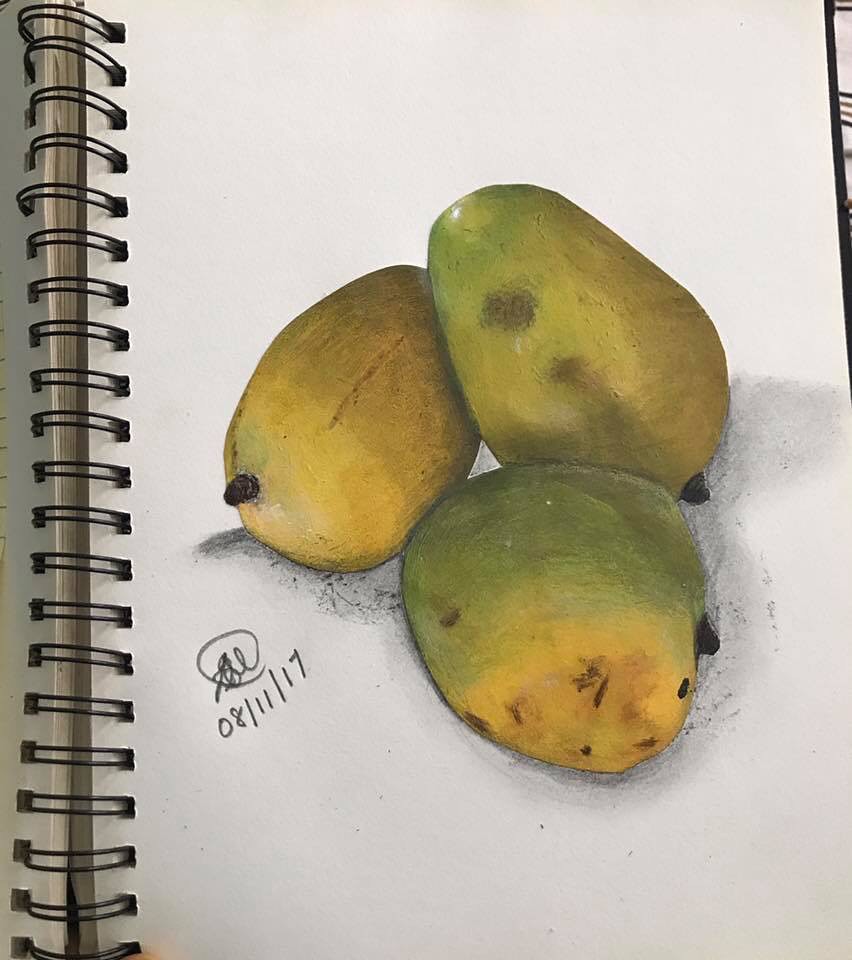A vibrant, detailed drawing captures three lifelike mangoes in rich, realistic colors on an open, spiral-bound tablet of paper. The page exhibits a signature, noted in a circular fashion, dated 08/11/17, inscribed in pencil. The artist skillfully uses shades of green, yellow, and orange to give the mangoes a three-dimensional appearance. Arranged in a seemingly random pile, the mangoes feature noticeable gray shadows beneath them, indicating a specific light source. Each mango is adorned with a black stem, while subtle imperfections, such as minor mars and bruises, add to their realism.